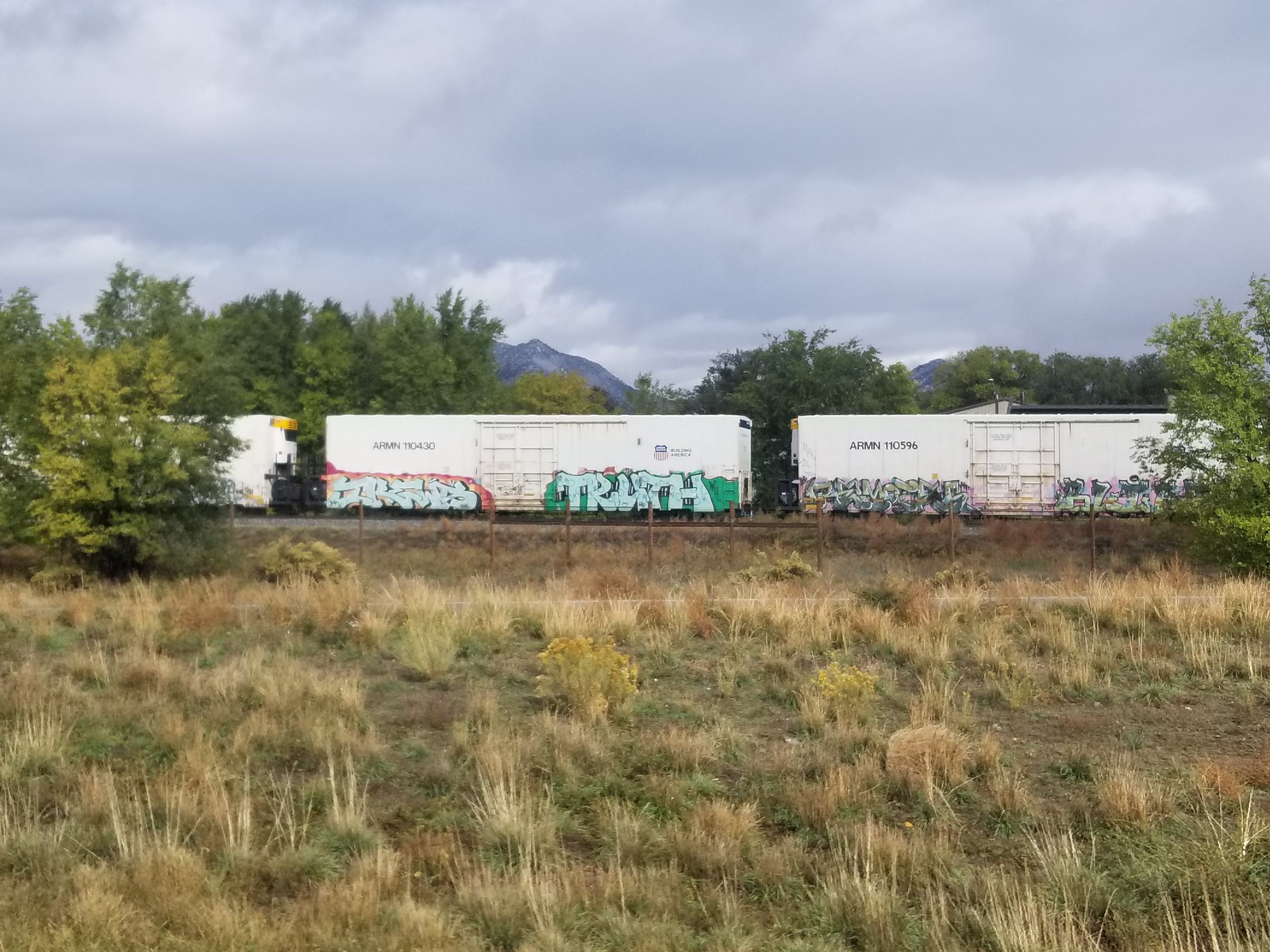This image captures a vibrant yet somewhat desolate scene of train tracks bisecting a dry, straw-colored field. Dominating the composition are three plain white train cars, each adorned with distinctive graffiti. The middle car stands out with two patches of colorful text: one has an illegibly pale-colored script set against a red background, and the other features the word "TRUTH" in light blue, bubbly block letters on a green background. The train car to the right also bears graffiti along its bottom edge, rendered in shades of gray and black, though the words are not legible. In the background, a line of deciduous trees and distant mountains rise under a canopy of gray, overcast sky, adding to the scene's somewhat muted atmosphere. The foreground is dominated by a mix of brown and green wild grasses, adding texture and depth to the photograph.